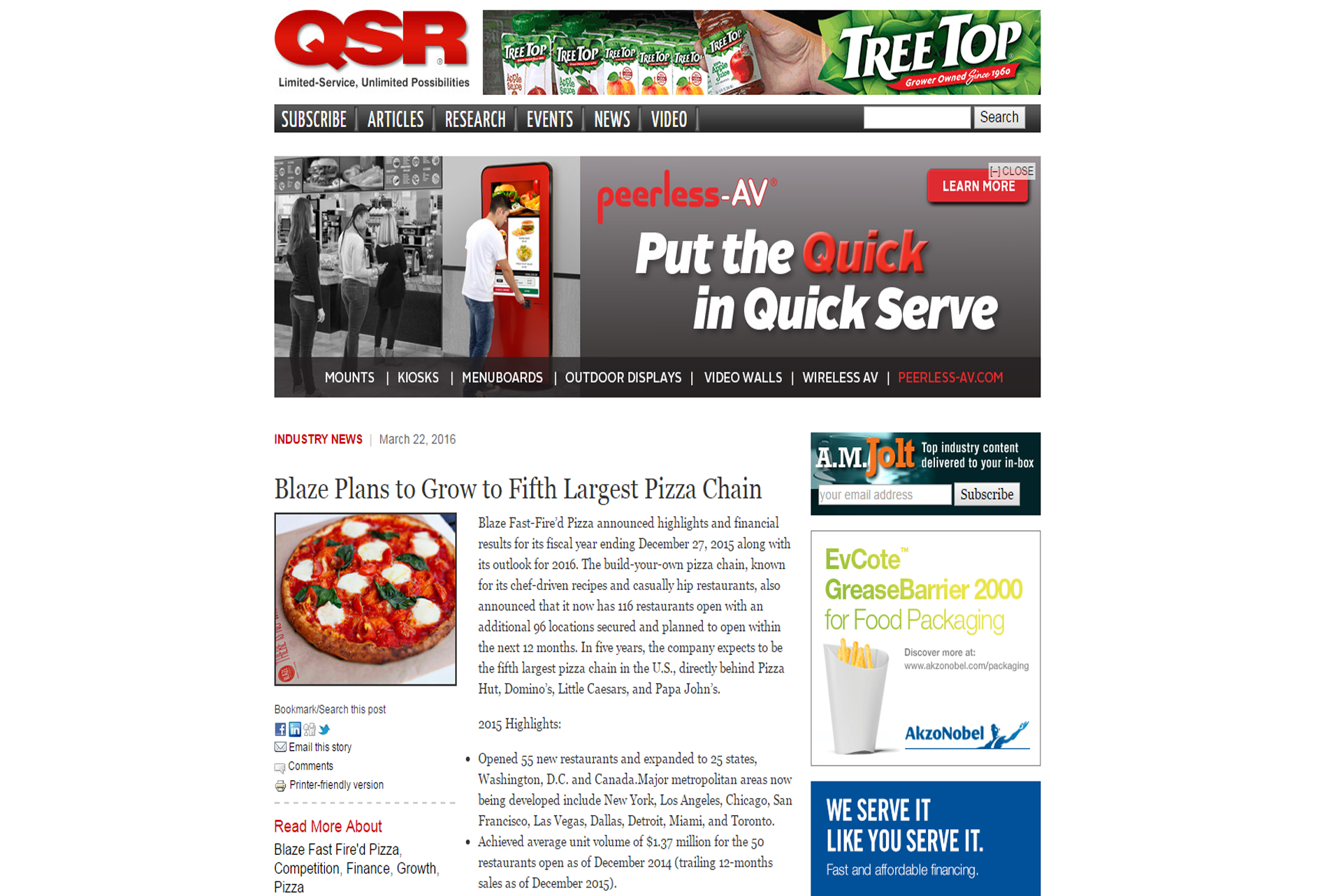The screenshot appears to be from a website named QSR, characterized by its distinct red capital letters in the upper left-hand corner. Below the QSR logo is the tagline "Limited Service, Unlimited Possibilities." Adjacent to this tagline is an advertisement for Treetop-branded boxed and bottled juices.

Beneath the ad, a navigation banner features various clickable text options that direct users to different sections of the website, including 'Subscribe,' 'Articles,' 'Research,' 'Events,' 'News,' and 'Video.' To the right of this banner, there is a search bar equipped with a search button.

The main body of the webpage prominently displays an article titled "Blaze Plans to Grow 5th Largest Pizza Chain," accompanied by an image of a Margherita pizza. The article details Blaze Fast-Fired Pizza's financial highlights and results for the fiscal year, focusing on notable developments within the food industry.